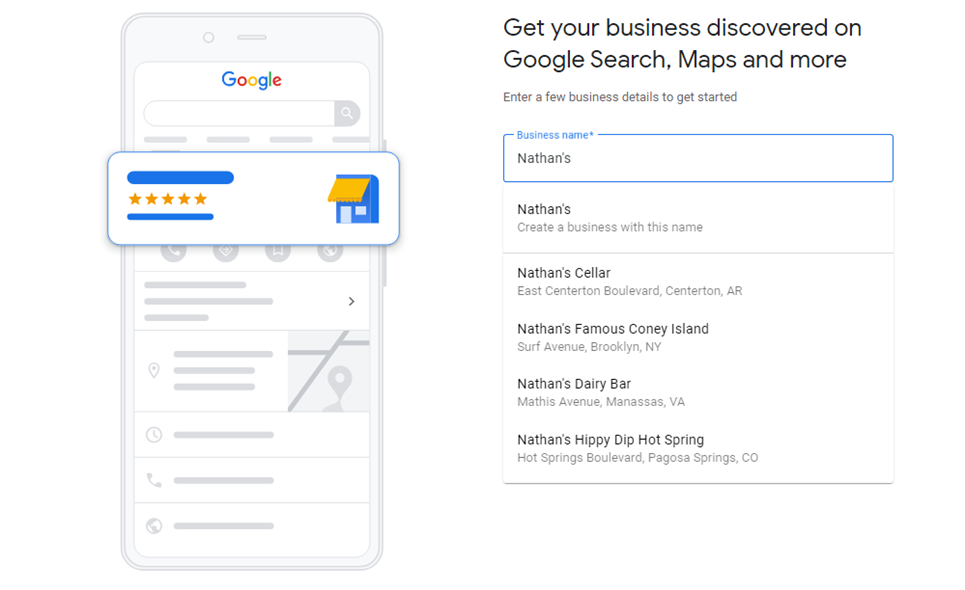This image is a screenshot demonstrating a Google business setup interface within a phone mock-up on the left side, accompanied by a form on the right. The phone mock-up displays a Google search page, featuring the iconic Google logo at the top, a search bar immediately below it, and a gray search icon. The image showcases a highlighted and enlarged section replicating a business entry mock-up. This highlighted portion includes a five-star rating layout on the left side, flanked by two blue borders—one above and one below. The entry also features an icon depicting a business with an overhanging yellow visor and a blue building facade.

To the right of the phone mock-up, the descriptive text header reads, "Get your business discovered on Google Search, Maps, and more." Directly below, instructional text encourages users to "Enter a few business details to get started." At the top of the form, the field for "Business Name" is highlighted, with the example "Nathan's" filled in. Following this, the prompt "Create a business with this name" is displayed. Further down, another entry reads "Nathan's Seller," accompanied by the business address: "East Centerton Boulevard, Centerton, AR."